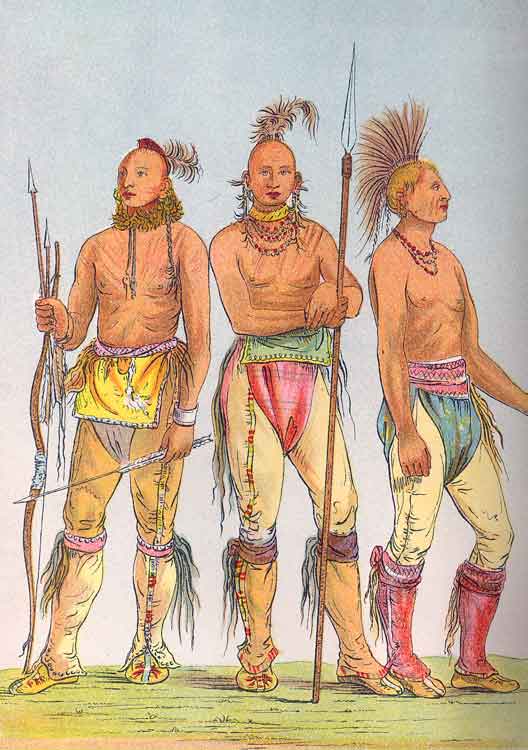This is a detailed drawing of three shirtless Native American men standing on a patch of green grass against a plain gray background. All three men have unique, creative hairstyles resembling mohawks, with one man's mohawk extending down his back. They are muscular and adorned with necklaces, with the man in the center additionally having dangling ear ornaments. On the left, the man has a bow and arrow, viewed from the front. He wears cream-yellowish pants and red boots. The central figure, who also faces forward, has his arms crossed while holding a spear and is dressed in tan pants with red and green accents and brown boots. The man on the right, who is seen in profile, also wields a bow and arrow and wears a wide necklace. His attire includes a gray belt, yellow chest covering, and gray underneath, with tan boots. The three men, appearing armed and vigilant, peer in different directions: left, right, and straight ahead.